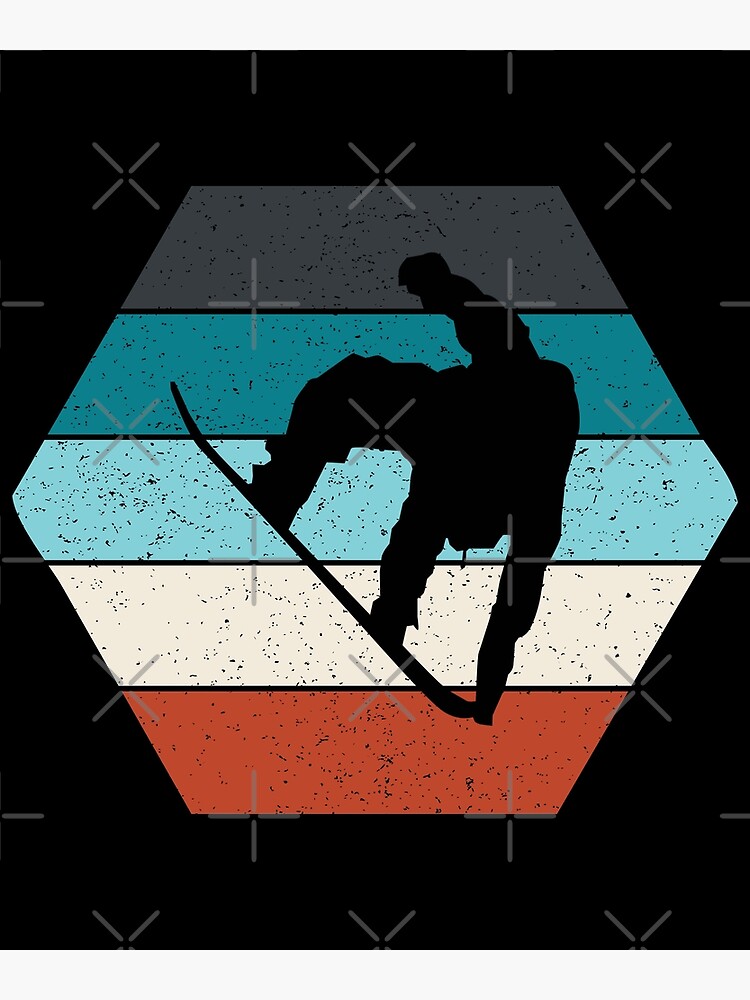A detailed graphic design displays a silhouette of a dynamic snowboarder performing an aerial trick. The snowboarder's silhouette is entirely black, with one hand gripping the front tip of the snowboard and the other hand raised mid-air, capturing a sense of motion and skill. The silhouette is prominently positioned within a central hexagon composed of five distinct, multi-colored stripes: a top dark grey stripe, followed by teal blue, light blue, beige with a yellow hue, and a bottom red stripe. These stripes feature small black dots that give a textured, marble-like appearance.

The hexagon is set against a deep black background that extends beyond its borders, emphasizing the central subject. Overlaying the entire image are translucent grey watermarks in the form of plus signs and multiplication signs. These symbols alternate in lines, adding a layered dimension that spans the entire image, contributing to the complexity and contemporary feel of the artwork.